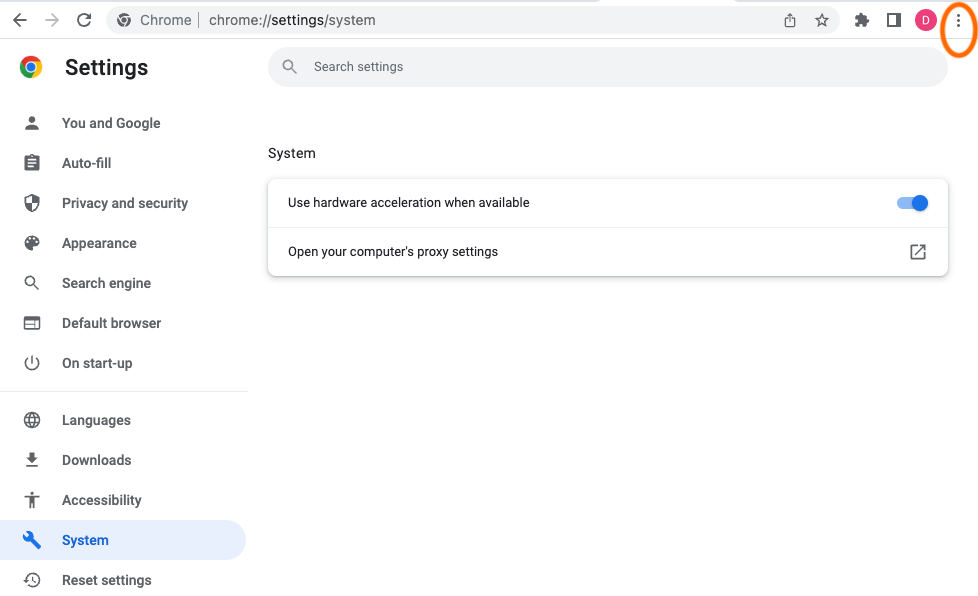This image is a detailed screenshot from the Google Chrome browser, specifically from the 'Settings' section under 'System'. The interface displays a clean white background with black text for easy readability. 

At the top of the image is the Chrome's address bar, which reads "chrome://settings/system", clearly indicating the current settings page being viewed. On the far right side of the address bar, there are three vertical dots encircled by an orange oval, commonly known as the "More" options menu.

On the left side of the screenshot, there is a vertical navigation menu featuring the Google Chrome logo at the top and a list of various settings categories. The categories listed are: Settings, You and Google, Autofill, Privacy and Security, Appearance, Search Engine, Default Browser, On Startup, Languages, Downloads, Accessibility, System, and Reset Settings.

The main section of the screen features a search bar labeled "Search settings", which is useful for quickly navigating to specific settings options. Below this, the heading "System" is displayed, indicating the current category being viewed. Under the "System" heading, there is an option labeled "Use hardware acceleration when available", which is toggled on, evidenced by the blue switch.

Just beneath this, there is another option labeled "Open your computer's proxy settings". This is accompanied by an icon suggesting that this option can be clicked for further actions or information.

The remainder of the page below these settings is blank, maintaining a minimalist design consistent with the white color theme of the screen.